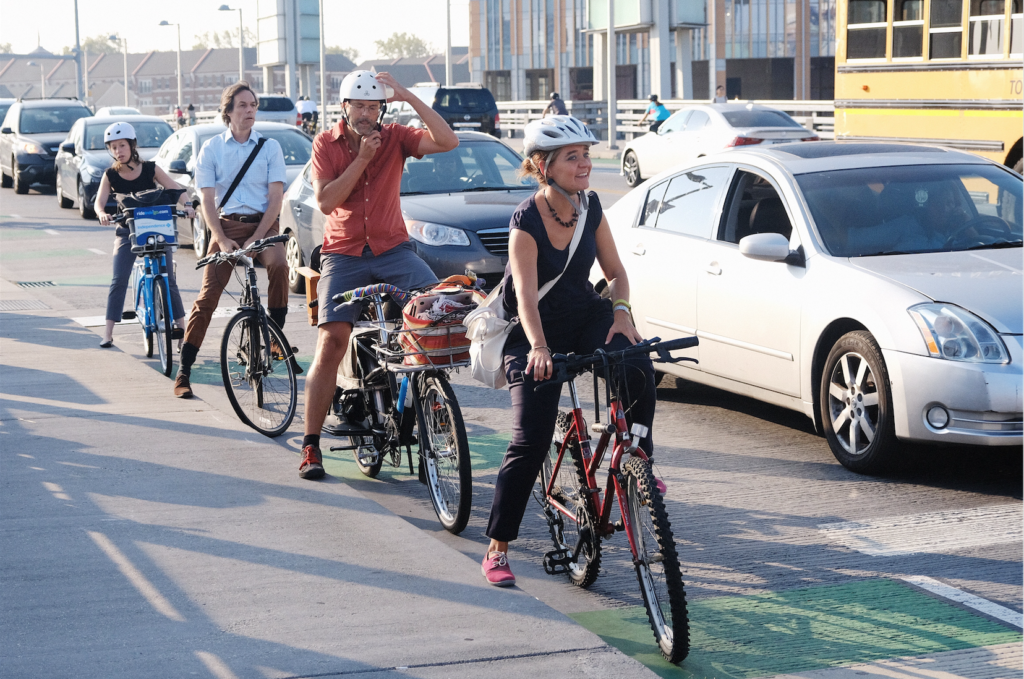In the bustling city street scene, four bicyclists occupy a bike lane adjacent to a row of five cars; all sedans except for the last one, which is a Range Rover. Behind the cars, the rear end of a yellow school bus is visible, partially cut off from the frame. The cyclists appear to be waiting at a stoplight, as evidenced by some riders resting their feet on the ground. The lead cyclist, a woman in an all-black outfit and white helmet, is smiling, while the man directly behind her, also donning a white helmet, appears more serious in a brown shirt and gray shorts. The third cyclist, another man without a helmet but dressed in semi-formal attire, has a basket with an orange handbag on his bike. The last cyclist, a woman in a black tank top and gray pants, wears a white helmet and completes the quartet. All of their bikes are predominantly black, with the lead woman’s bike featuring bluish accents. The scene is set on what appears to be a concrete road with green bike lane markings, amidst a backdrop of blurred city buildings and green trees under a hazy sun.